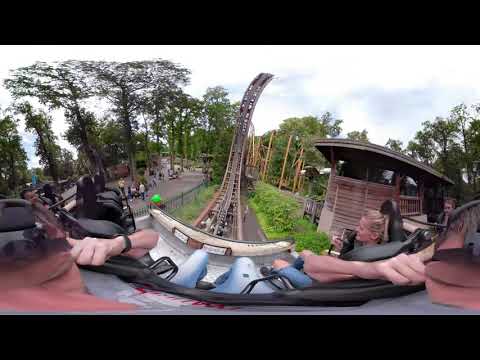The image, captured with a 360-degree or ultra-wide lens, depicts an action scene viewed from the back car of a roller coaster. The scene is set during the day, and the roller coaster track can be seen descending 20-30 feet before shooting straight up into the air in the center of the image. Below, the bottom third of the image features seats with distorted legs, arms, and hands of passengers strapped in, ready for the ride. 

On the right side, there's a wooden shack which appears to be the loading area for the coaster, with a younger blonde woman standing nearby, looking out. Additionally, the image reveals people standing around the area, possibly waiting for their turn or observing. In the background to the left, there are four to five tall trees and various greenery, including bushes, adding a natural element to the scene. 

The photograph also includes a detailed view of two people at the base of the image, likely the photographer and a companion, providing a point-of-view experience. Overall, the presence of trees, green areas, and a crowd of people walking around creates a lively, immersive atmosphere.